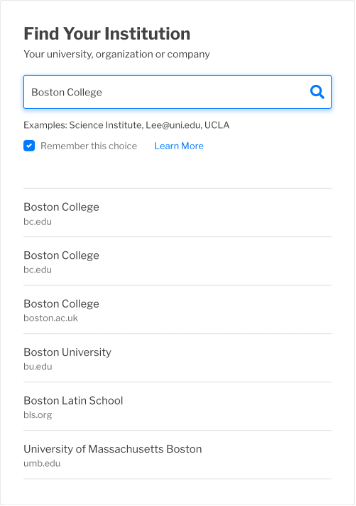A user is typing in a search box to find their institution. The search term currently entered is "Boston College." Below the search box, the interface provides example suggestions, such as "UCLA," to assist with the search. There's an option with a blue checkmark labeled "Remember this choice" to save the selected institution in case of computer crashes.

To the right of the search bar, there is a link labeled "Learn more" in blue. Multiple results for "Boston College" appear, including variations like "Boston College - bc.edu," "Boston College at boston.ac.uk," "Boston University - bu.edu," "Boston Latin School," and "University of Massachusetts Boston."

The interface is simple, with a white background. The search box is outlined with a blue border, and the magnifying glass icon within the box is also blue. The text "Find your institution" is bold, making it stand out slightly more against the otherwise plain design.